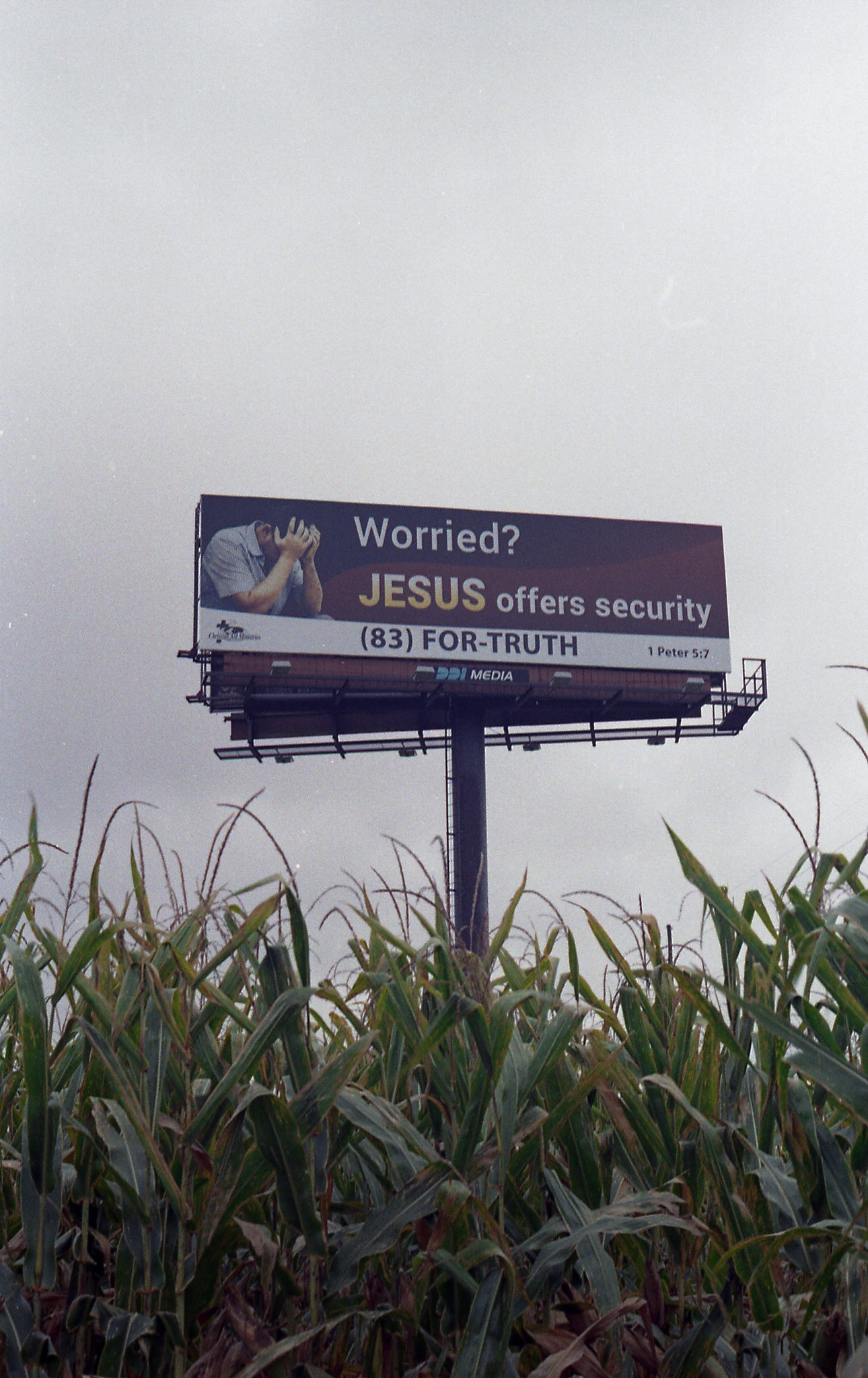This photograph captures a billboard standing in the middle of a dry, brown field of what appears to be corn stalks and weeds, hinting at a winter or late autumn setting. The scene is framed by an overcast, uniformly gray sky, adding a somber tone. The billboard, mounted on a high pole, prominently features a man wearing a short-sleeved blue shirt, his head bowed into his hands, conveying a sense of overwhelming stress or grief. Set against a black background, the text in white letters reads, "Worried?" followed by "Jesus offers security" in a combination of yellow and white lettering. Below this, a white banner displays the phone number "(83) 4FOR-TRUTH" and the Bible verse "1 PETER 5:7." Additionally, the structure beneath the billboard bears the word "MEDIA" in white letters, preceded by some stylized letters that are not fully legible. An indistinct cross also appears, possibly indicating a religious affiliation or church sponsorship. The overall composition of the photo, from the dry, lifeless vegetation to the gray sky, underscores a mood of desolation and concern.